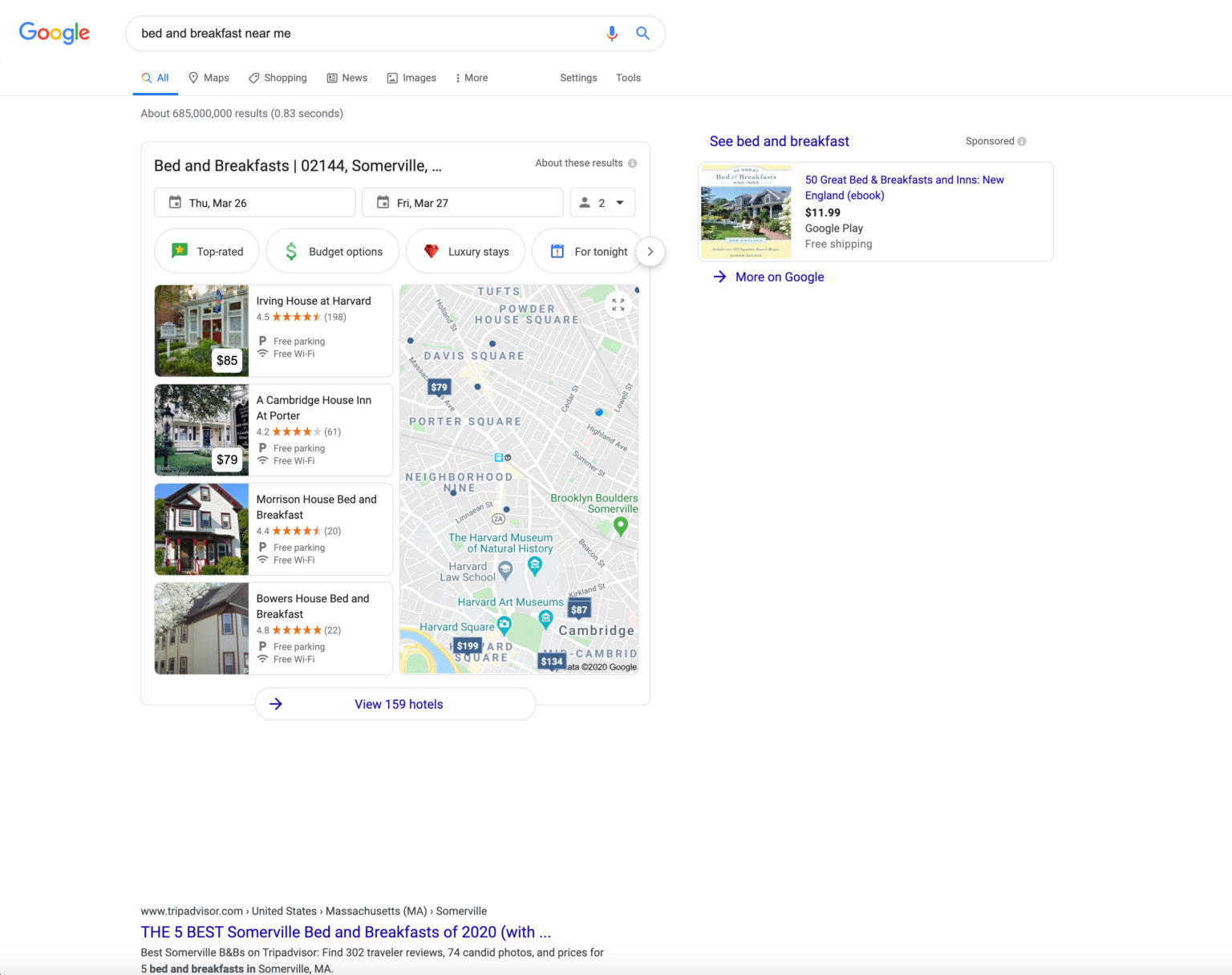The screenshot captures a Google search page displaying results for "bed and breakfast near me" within the zip code 02144. The user has specified their stay dates as Thursday, March 26, to Friday, March 27, for two people. Various filters are available, including options for top-rated, budget, luxury stays, and bookings for tonight. The search results showcase several bed and breakfast options:

1. **Irving House at Harvard** - Priced at $85 per night with a rating of 4.5 stars.
2. **A Cambridge House Inn at Porter** - Available for $79 per night with a rating of 4.2 stars.
3. **Morrison House Bed and Breakfast** - Boasting a rating of 4.4 stars.
4. **Bowers House Bed and Breakfast** - Top-rated at 4.8 stars.

A button at the bottom invites users to view an additional 159 hotel options. A map on the right-hand side shows the locations of these bed and breakfasts.

Additionally, there is a sponsored ad on the right side of the page for an e-book titled "50 Great Bed and Breakfasts in New England," available on Google Play for $11.99 with free shipping. A link to TripAdvisor can be found at the bottom of the page, likely offering further reviews and travel information.